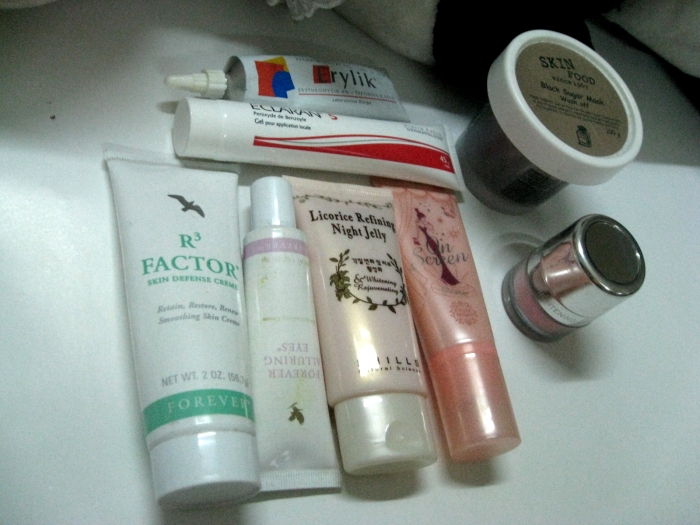On a pristine white countertop, a collection of skincare products is carefully arranged, each distinct yet unified by a theme of elegance and functionality. Dominating the center is a white squeeze tube of R3 Factor Skin Defense Cream, adorned with a bird logo and green lettering, capped by a sleek white lid and exhibiting a shiny surface.

Adjacent to it is another tube bearing the same bird logo, differentiated by its purple stripe and matching purple lettering; however, the exact text remains unreadable. Further along the lineup is a pink tube of night jelly for facial application, identified by its black lettering and glossy finish. Next in line is another pink tube, slightly squished, rendering its text illegible.

Towards the top of the arrangement sits a red-and-white tube, distinct yet cohesive with the rest of the collection, and just above it is a metallic tube characterized by a pointed nozzle, suggesting precision in application.

On the far right side, a sophisticated black jar with a white lid and a gold label stands out, hinting at a luxurious night cream, the word "skin" faintly discernible on its surface. Finally, another tube features a silver, shiny top, revealing a pink substance within, completing this curated assembly of skincare essentials.